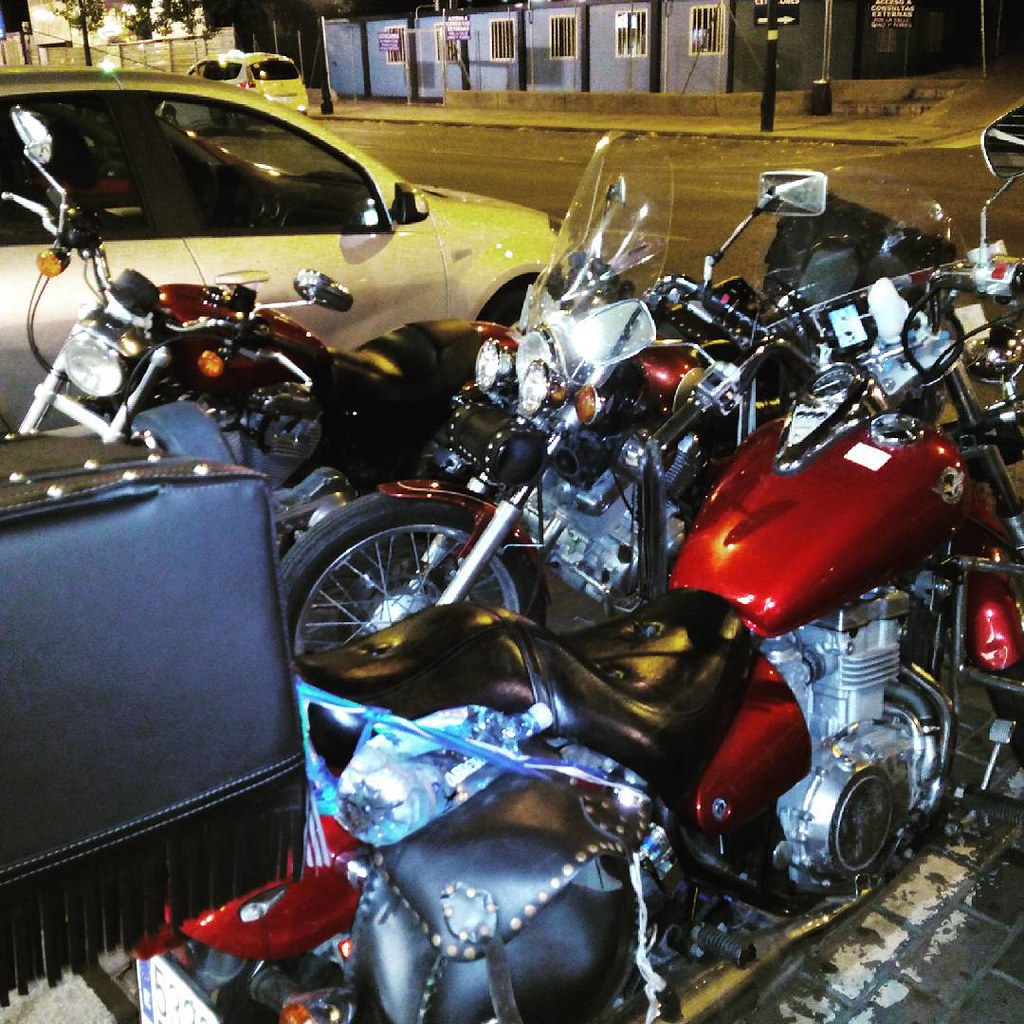This nighttime photograph, shot in color and in a square format, prominently features three chopper-style motorcycles, evoking the essence of Harley-Davidsons. The scene is somewhat zoomed in, creating an intimate but cluttered view of the vehicles. The motorcycle in the foreground boasts a red gas tank, black leather seat, chrome motor, and standard side mirrors. It also features a black leather mount with tassels and is positioned facing a road to the right of the photograph. Another motorcycle, also with a red tank, metal mirrors, and a front light, is oriented to the left. The third motorcycle, distinguishable by its glistening white lights, black wheels, and black seat, also faces leftwards.

A silver car, potentially a hatchback, is visible in the top left corner facing the top right. There's an additional vehicle, described variably as a yellow cab and an off-colored yellow car, also on the left side of the image, featuring dark tinted windows. Street lights illuminate the scene from above, casting a clear, focused light on the subjects. In the background, there's a flat, blue building with five windows framed with security bars, adding a rustic urban backdrop to this snapshot of nighttime vehicular rest.